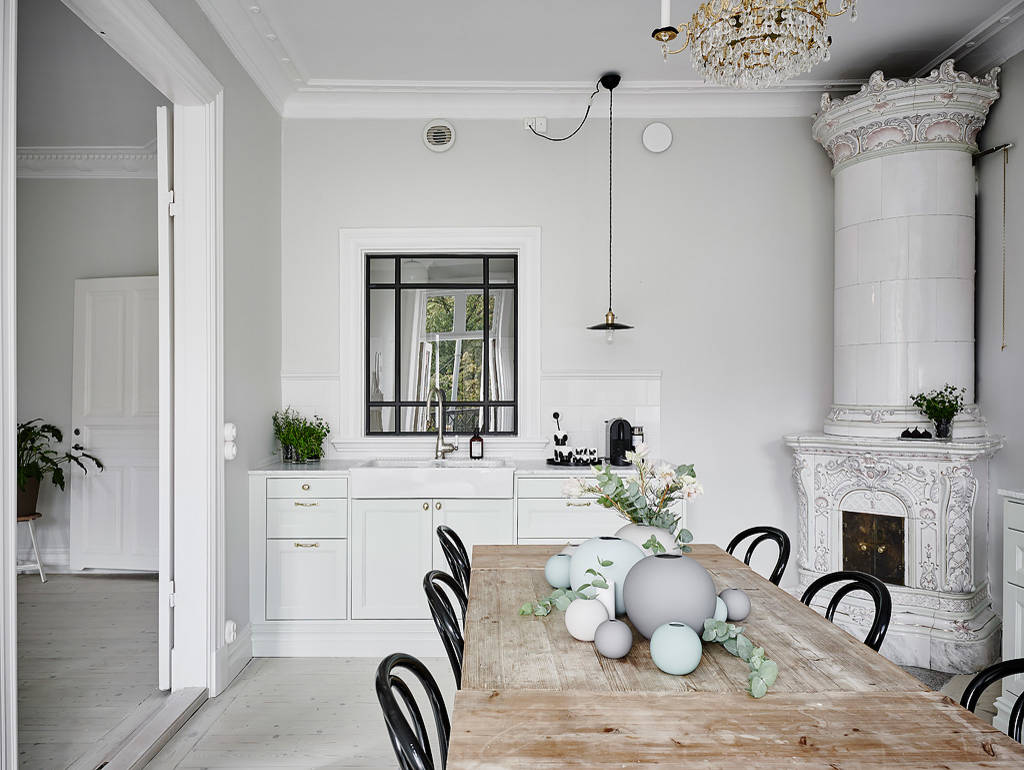The image depicts a bright and impeccably clean kitchen-dining room with a predominantly white color scheme, radiating a sense of purity and modernity with a hint of country chic flair. The walls, floors, and ceiling are all white, enhancing the room's fresh and airy atmosphere. Dominating one corner is a grand, white furnace or stove, featuring an ornate, embossed design and decorative crown molding at the top. This elaborate structure stands out with its rounded upper section, contributing to the room's elegant yet homely vibe.

Central to the room is a long, light wooden farm-style table adorned with assorted round ceramic vases filled with eucalyptus, exuding a rustic charm. Surrounding the table are sleek black chairs, providing a striking contrast to the room's predominant whiteness. Directly ahead, a large window sits above a simple, unadorned white sink and countertops, flanked by white cabinets and drawers for a streamlined look. 

Additionally, a pendant light hangs stylishly over the sink area, illuminating the space. Adjacent to the sink, a white cupboard houses more kitchen essentials, including a coffee machine, adding functionality to the room. To the right of this setup is a white, elaborate fireplace, further blending modern design with classical elements. This harmonious blend of minimalist and ornate details defines the character and aesthetic of the room.